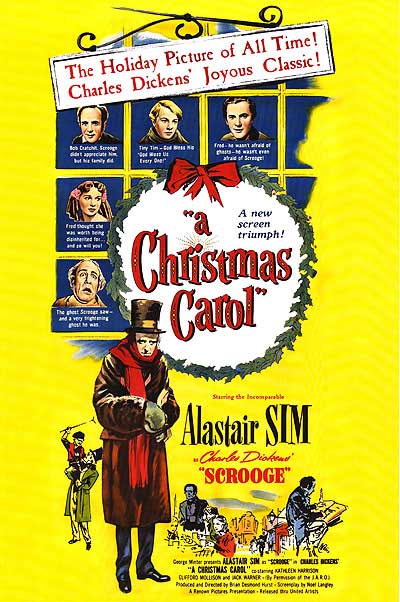The image is a vintage poster for a film adaptation of Charles Dickens' "A Christmas Carol." It is rectangular, measuring approximately four inches in height and three inches in width, with a bright yellow background. At the top, there is a tilted metal sign hanger, with the right-hand side of the sign being higher than the left. The sign itself is also rectangular with a white background and red print, reading, "The Holiday Picture of All Time, Charles Dickens, Joyous Classic."

Central to the design is a prominent Christmas wreath outlined in green with a red bow at the top, enclosing a white circle where the title "A Christmas Carol" is displayed in red print, followed by the black text "A New Screen Triumph." Below, an illustration features key characters from the story, including Scrooge, Tiny Tim, Bob Cratchit, and others, rendered in a drawn style indicative of an artistic adaptation rather than photographs. 

In a grid formation above the wreath, there are small illustrated headshots of the characters, including Bob Cratchit on the top left, Tiny Tim in the center, and other figures such as Fred and one of the ghosts, though the details are less clear. The names Alistair Sim and Charles Dickens are highlighted at the bottom in black and red text, respectively, indicating the lead actor and the author. The overall aesthetic suggests a nostalgic and classic portrayal, emphasizing the timeless appeal of the story.